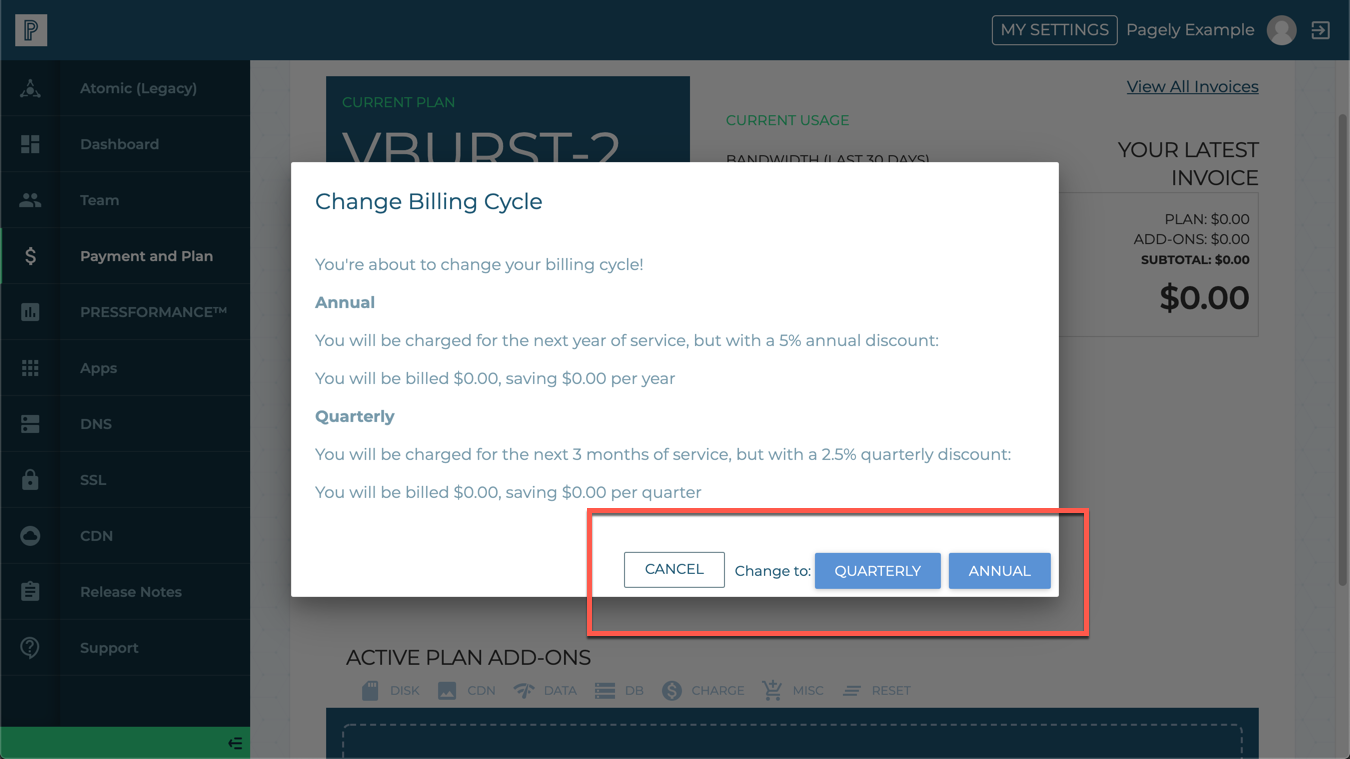The screenshot displays an invoice interface titled "My Settings - Pagely Example" related to the "Current Plan B: Burst 2." On the left-hand side, there's a vertical navigation panel with the following menu options: Atomic Legacy, Dashboard, Team, Payment and Plan (highlighted), Press Formants, Apps, DNS, SSL, CDN, Release Notes, and Support.

In the center is a pop-up overlay titled "Change Billing Cycle." Behind this pop-up, the latest invoice details are visible, showing "Plan 0, Add-on 0, Subtotal 0." The pop-up message informs the user that they are about to change their billing cycle. It provides two options: 

1. **Annual:** Indicates that the user will be charged for the next year's service with a 5% annual discount, resulting in zero cost and zero savings per year.
2. **Quarterly:** Indicates that the user will be charged for the next three months of service with a 2.5% quarterly discount, resulting in zero cost and zero savings per quarter.

At the bottom of the pop-up are three buttons: "Cancel," "Change to Quarterly," and "Change to Annual."